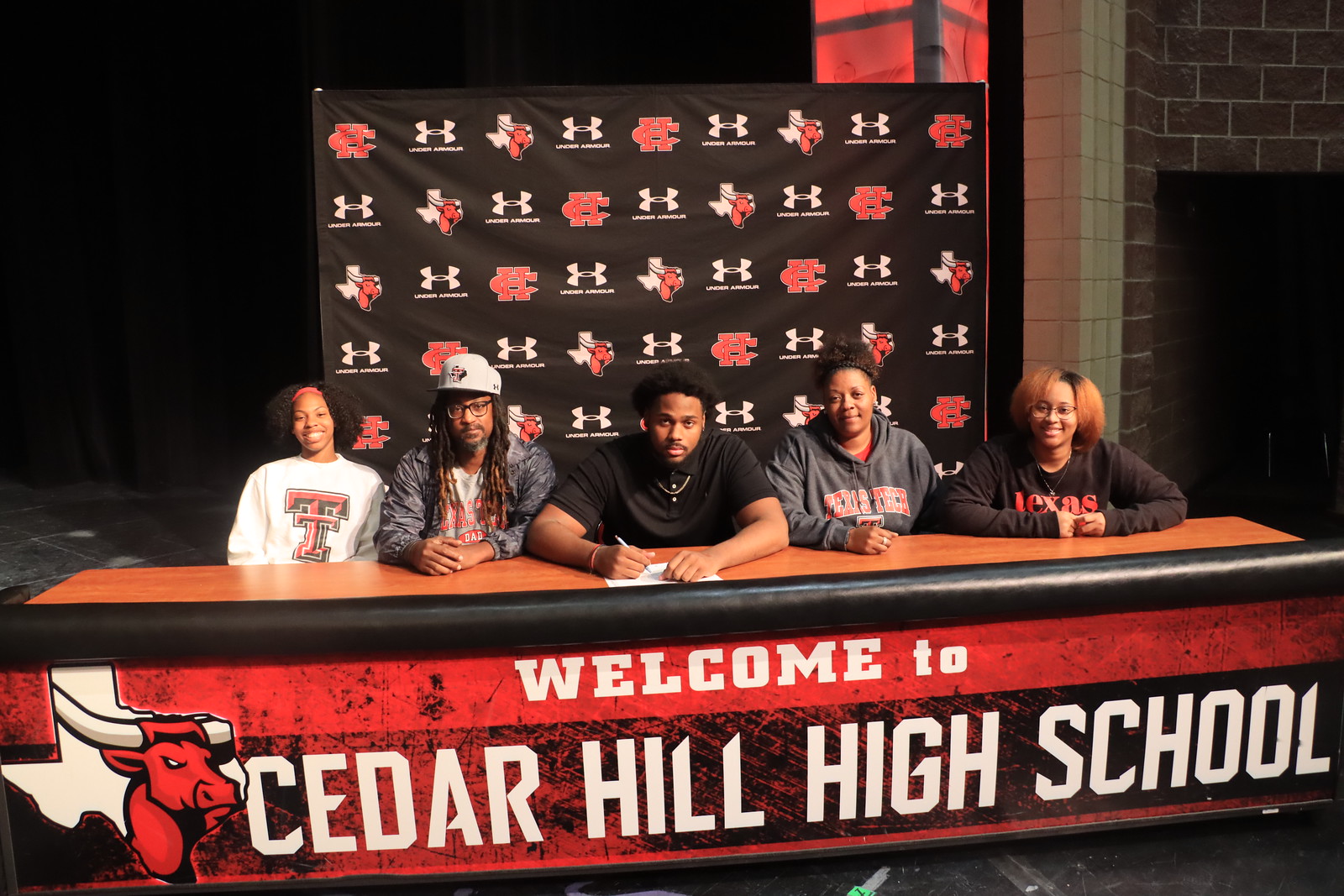This is a photo of five young African American adults—three women and two men—sitting behind a long, rectangular table in what appears to be a formal gathering. The table is adorned with a prominently displayed red and orange banner that reads "Welcome to Cedar Hill High School" in white letters. On the left side of the banner, there is an image of the state of Texas with a red bull featuring white horns. The table behind which they are seated has a black front, and there's a symbol of Cedar Hill High School in the backdrop. This backdrop is black and covered with an array of white Under Armour logos as well as the school’s emblem—a red bull over the outline of Texas and the overlapping letters "CH." The scene suggests a significant event, possibly a signing ceremony, given the presence of a piece of paper in front of one of the men, indicating he might be committing to a future endeavor while his family watches supportively.